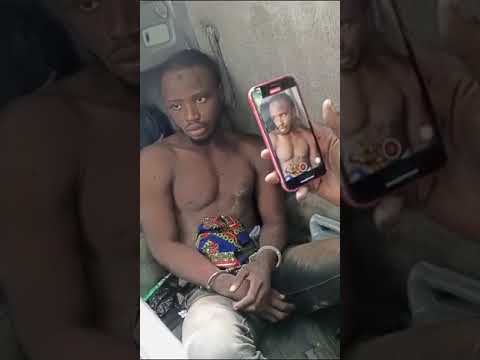This color photograph, presented in portrait orientation, showcases a young African-descendant man with medium brown skin and short black hair, sitting shirtless against a gray cement outdoor wall. His arms are crossed in front of his lap, holding a brightly colored fabric that features a mix of purple, pink, yellow, blue, and red patterns. He appears to be wearing light gray blue jeans, visibly covered in dirt. The scene includes a hand extending from the right, holding a smartphone with a pink case, capturing an image of the seated man. This photograph is embedded within a larger, darkened landscape orientation print of the same image, with the left third showing an enlarged section of the man's upper torso and face, and the right third highlighting an up-close image of the smartphone and hand. Notably, the man is in handcuffs, which are causing his crossed arm position in his lap. This detailed composition, blending representational elements, evokes a powerful sense of atmosphere and narrative.